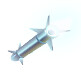This is an incredibly small, blurred thumbnail image of a metallic, torpedo-like spaceship set against a white void background. The spaceship is angled downwards towards the lower left, resembling it's descending back to Earth. The body of the spaceship is cylindrical with a classic chrome shading, giving off a shiny, silver appearance. At the top end, the spaceship has three antenna-like spikes—two on top and one on the bottom. Meanwhile, the bottom end features four fins arranged in an X-formation, ending in what appears to be an opening emitting a bright white light. Despite the blurry nature of the image, the intricate details like the spikes and the X-shaped fins are discernible, adding to its complex design.